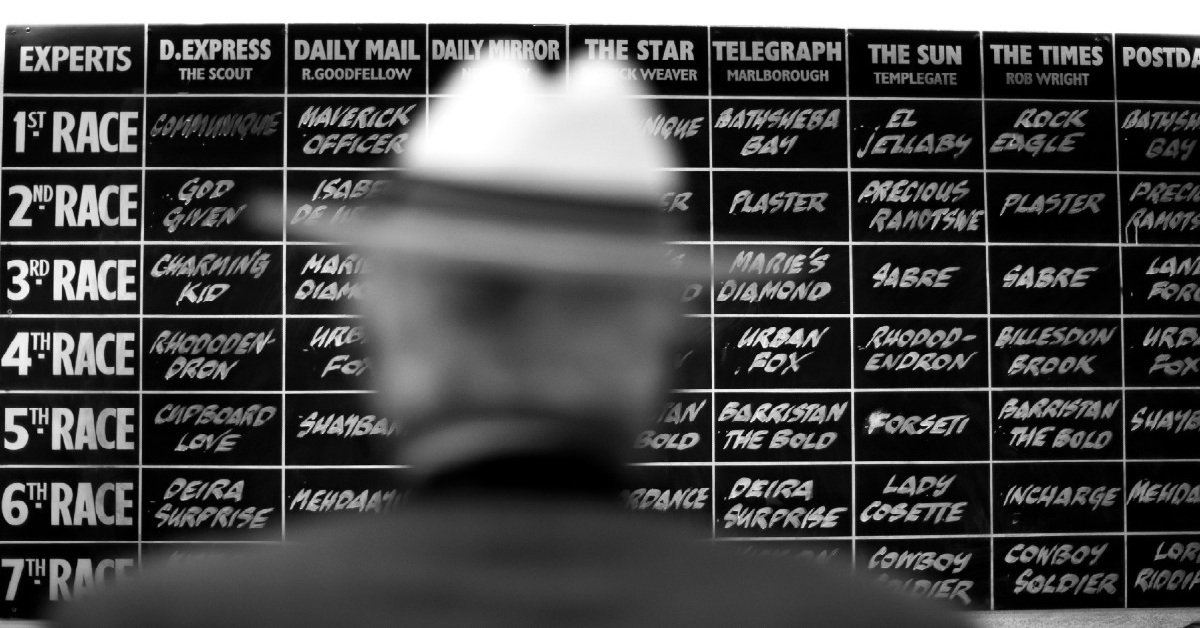The photograph captures the blurred silhouette of a man wearing a white hat and a dark-colored suit, with grayish hair, standing close to a blackboard that details horse race predictions. The blackboard is arranged like a grid or spreadsheet, clearly visible despite the man obscuring portions of it. At the top of the columns are names of newspapers and experts, including D-Express, Daily Mail, Daily Mirror, The Star, Telegraph, The Sun, and The Times. Down the left side are rows labeled for different races: first race, second race, and so on through the seventh race. Each cell within the grid contains handwritten names of horses predicted to win each race, such as God Given, Charming Kid, Rhododendron, Maverick Officer, Bathsheba Bay, and Plaster. The image is in black and white, emphasizing the contrast between the clear details of the blackboard and the blurred figure of the man standing in front of it.